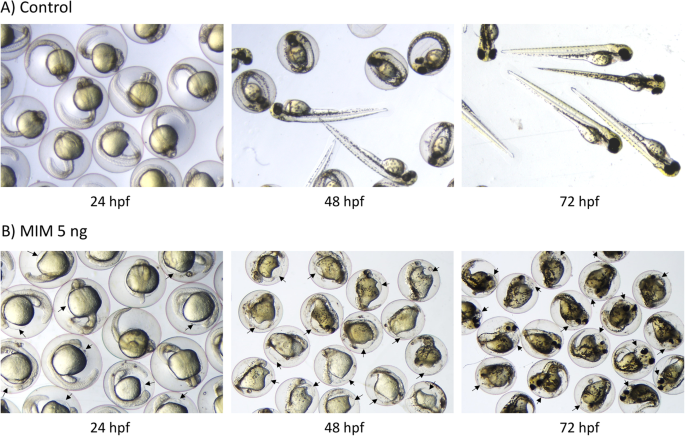The landscape-orientation image is a scientific visual aid comprising two rows, illustrating the developmental stages of fish embryos under a control condition and a treatment (MIM5NG). The top row, labeled "A Control," and the bottom row, labeled "B MIM5NG," each consist of three photographs. 

Both rows depict embryos at three specific time points: 24 HPF (hours post-fertilization), 48 HPF, and 72 HPF. In the control row, the 24 HPF image shows translucent egg spheres with light greenish, tadpole-like embryos inside. By 48 HPF, some embryos have started to emerge, exhibiting elongated bodies. At 72 HPF, all embryos have hatched, displaying longer bodies with prominent dark eyes.

Conversely, in the MIM5NG row, all embryos remain confined within their translucent eggs across all three time points. At 72 HPF, arrows indicate the presence of some kind of sack inside the eggs, highlighting a potential developmental anomaly or delay caused by the treatment. These detailed photographs emphasize the differences in developmental progression between the control and treated groups over time.